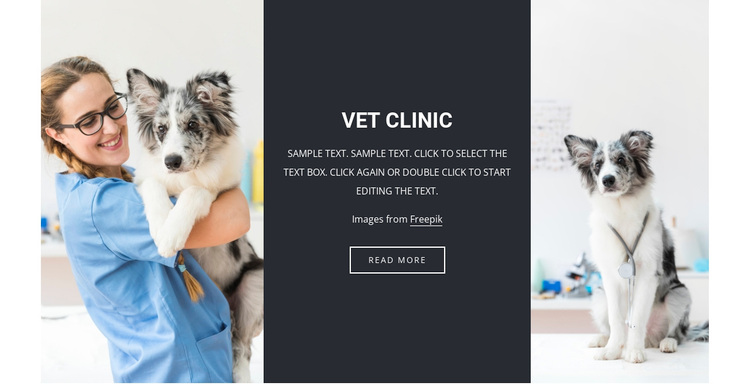In the image, the left side features a light gray background with a lady prominently standing. She wears a blue, short-sleeved jacket and has long, light brown braided hair. Sporting glasses, she's holding an adorable black and white dog with predominantly white fur underneath and a mixed black-and-white face. Centrally, a large gray text box with white print reads: "Vet Clinic, Sample Test, Sample Test," accompanied by instructions to edit the text. Below this, the source "Images from Free Pick" is referenced with an underline. A small white square within the text box states, "Read More," in gray print. On the right side of the image, the same black and white dog is seen sitting upright on its hind legs in front of a white wall, backed by a small shelf. The floor beneath is also white. The shelf holds a few blue items, one resembling a cell phone. The dog wears a white rope collar with tags.